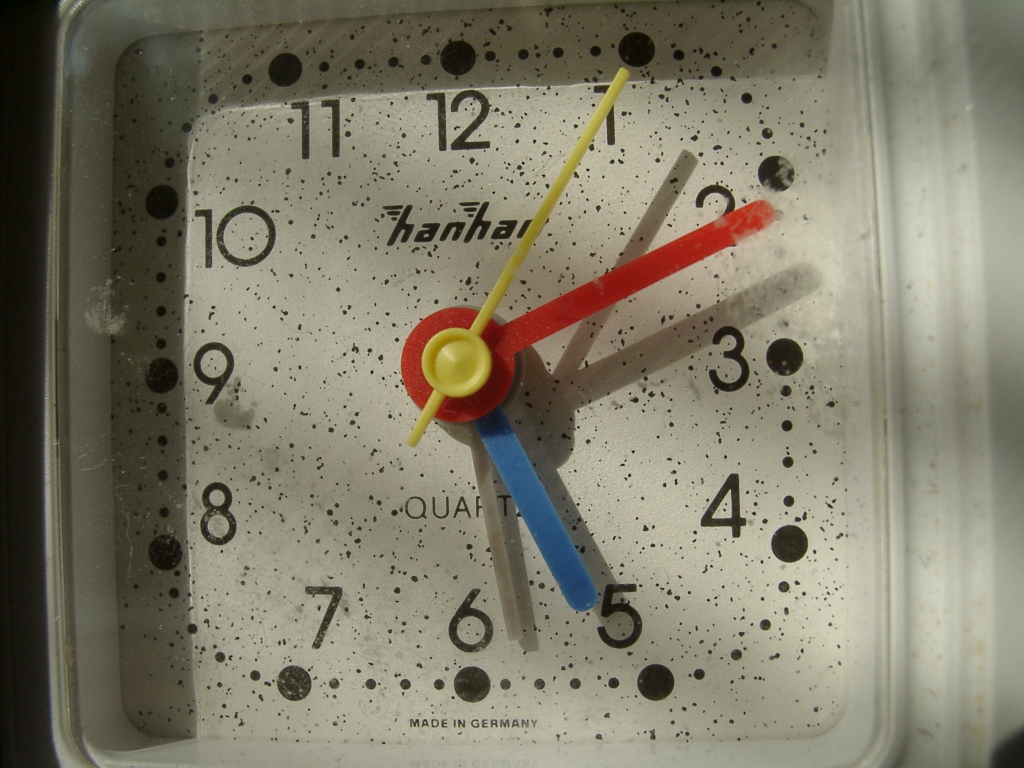This image captures a square-shaped, vintage-style analog clock with a predominantly simple design. The clock face, which is mostly a faded white, features a scattered or splattered pattern of black and gray specks. Surrounding each of the black numerals from 1 to 12, there are large black dots, with smaller black dots marking the minutes between each numeral. The clock hands are notably colorful and plastic-looking: the second hand is a long, skinny yellow, the minute hand is solid red, the hour hand is light blue, and there is an additional gray hand that appears next to the blue hour hand, whose purpose is unclear. Above the center of the clock hands, the name "Han Han" (H-A-N H-A-N) is displayed, indicating the clock's maker. Beneath the hands, the word "Quartz" is printed, and at the very bottom, below the six, the text "Made in Germany" is present. The clock is encased in a silver-colored metal border with a glass pane covering the face.